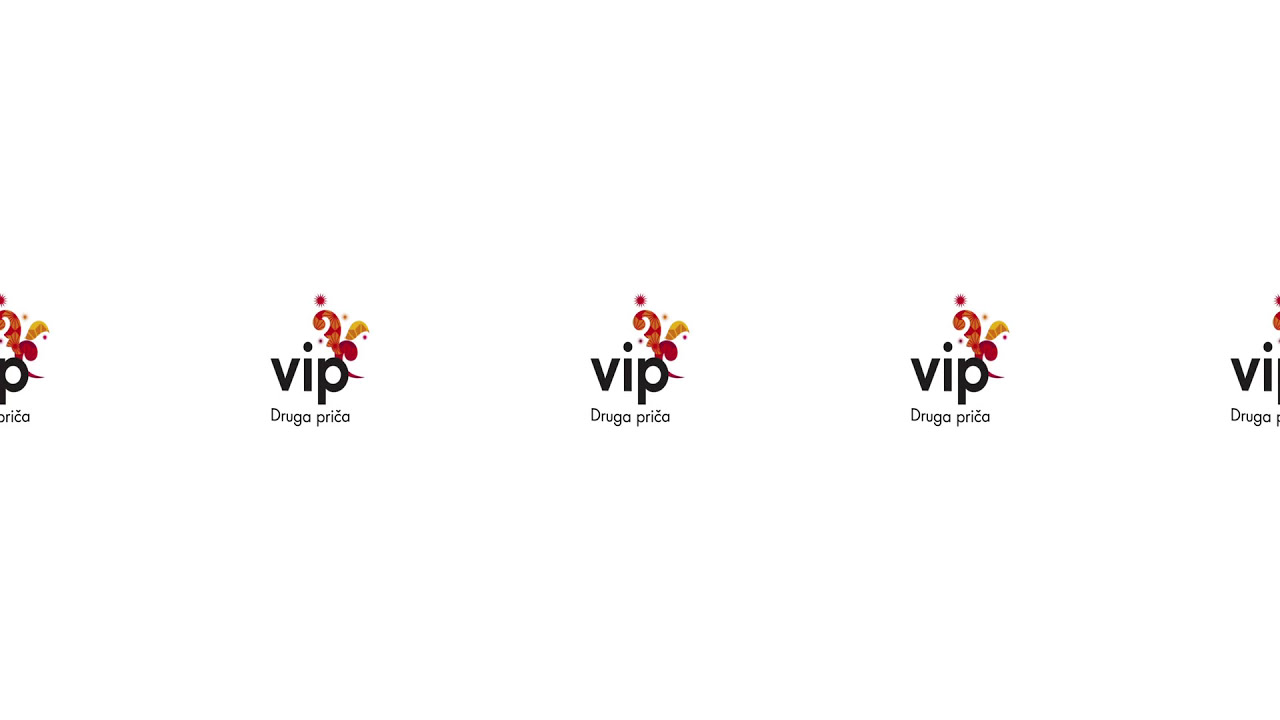The image features a repeating pattern of the text "VIP Druga Prica" in black lowercase letters on a white background. This phrase is repeated five times horizontally across the image, with evenly spaced intervals. Notably, the first instance of this pattern is cropped, showing only the letter "P," followed by "risa," due to the cut-off "P." Similarly, the last pattern is partially displayed, showing "V-I" and a partially visible "Druga." Above each instance of "VIP Druga Prica," there is a decorative red emblem with yellow and gold elements, including what appears to be a gold feather and pink dots, possibly resembling a heart shape above the "C" in "Prica." The decorations also include swirlies and curves that add a touch of elegance to the design.